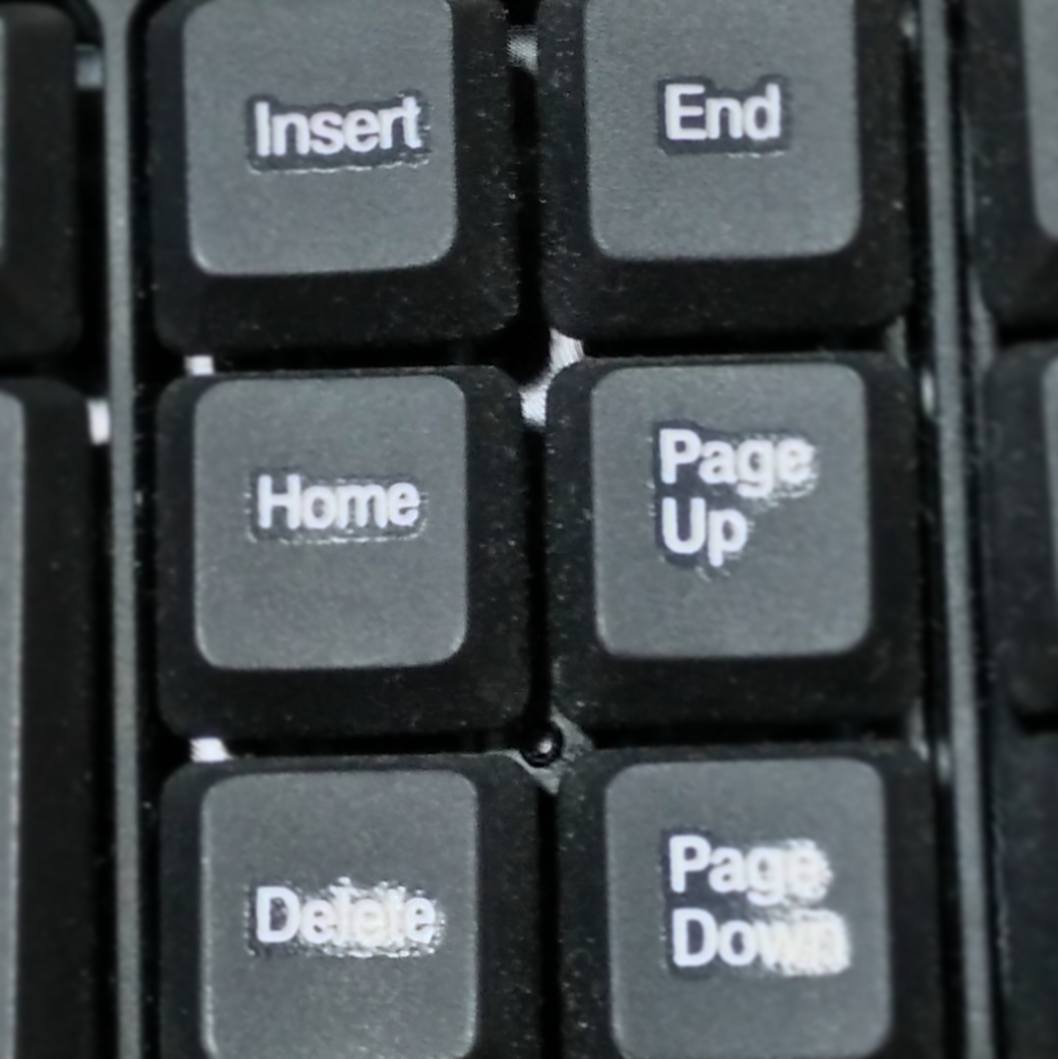This image is a close-up of a section of a black desktop keyboard, focusing on the numpad area. The photo captures six distinct keys with white lettering, which are arranged in three rows. The top row features the "Insert" button on the left and the "End" button on the right. The middle row includes the "Home" button on the left and the "Page Up" button on the right. The bottom row consists of the "Delete" button on the left and the "Page Down" button on the right. The keyboard appears raised with visible metallic bits between the keys, suggesting it is an older or less expensive model, possibly with sticker-like labels on the keys, often found in desktop setups. Additionally, portions of adjacent keys are visible on the left and right sides, hinting at a broader keyboard layout beyond the cropped frame of the image.